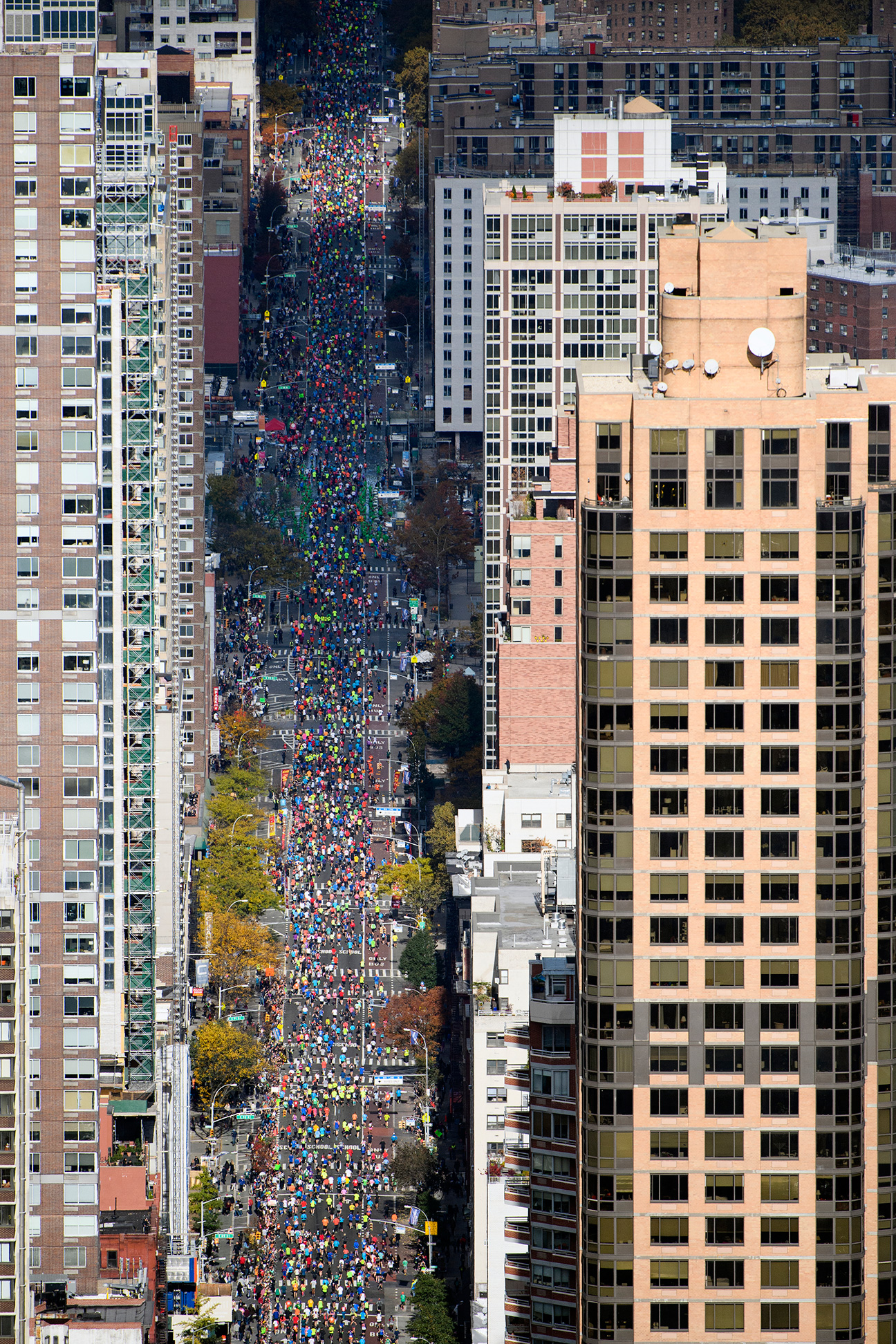The image captures a bustling, aerial view of a wide city street nestled between towering skyscrapers, some of which are over 20 stories high with numerous windows. The perspective suggests it was taken from a high vantage point, possibly from a helicopter. The street, devoid of traffic, is packed shoulder-to-shoulder with people wearing colorful outfits in every hue imaginable—yellow, red, green, blue, and more. The scene suggests a large-scale event like a marathon or a march. The people appear like tiny, multicolored dots due to the altitude. Lining both sides of the street are autumnal trees adorned in shades of orange, yellow, and red, indicating the season. The buildings close to the foreground have a distinct pink hue, possibly apartment complexes or business offices. The sunlight casts varying shadows over the throngs of people, with sections shaded by the skyscrapers while other parts are bathed in sunlight, enhancing the dramatic effect of the scene.